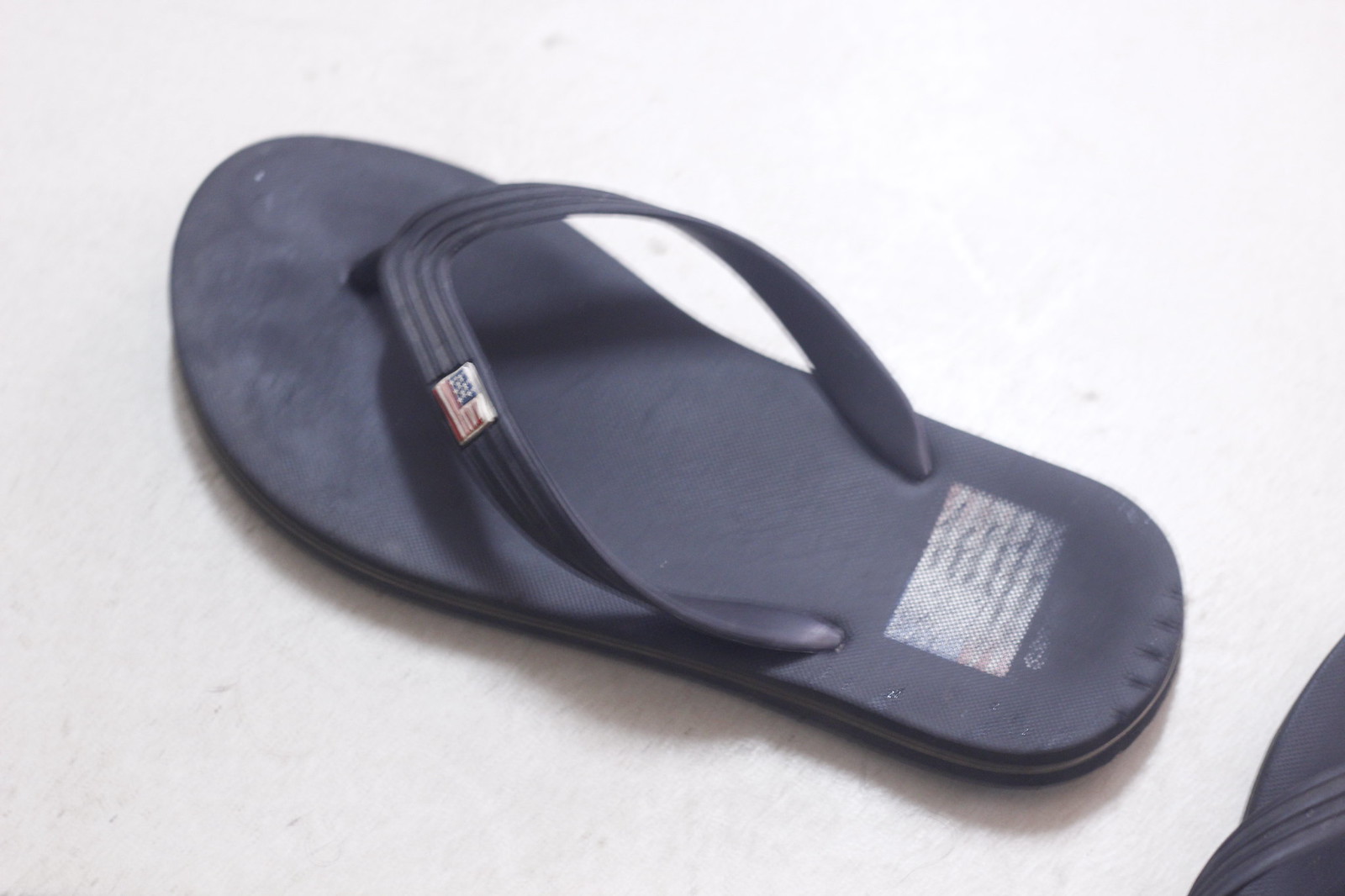The image is a detailed photograph of a well-worn thong-style sandal resting on what appears to be a rough-textured concrete surface. The sandal is primarily blue and has a distinctive design featuring a central strap that bifurcates into two additional straps, wrapping to the sides of the foot. Prominently, one of the straps bears a small emblem resembling the American flag. A similar rectangle, once vividly depicting an American flag, is found on the heel area, though it is now heavily faded, blending into a more uniform white from extensive use. At the top of the sandal, the indentations of the wearer's toes are distinctly visible, indicating frequent use. The footwear's partner can be glimpsed in the bottom right corner of the photograph, though mostly cropped out of the frame. The overall scene is set against a flat, concrete background, highlighting the stark contrast between the worn blue sandal and its rugged resting place.